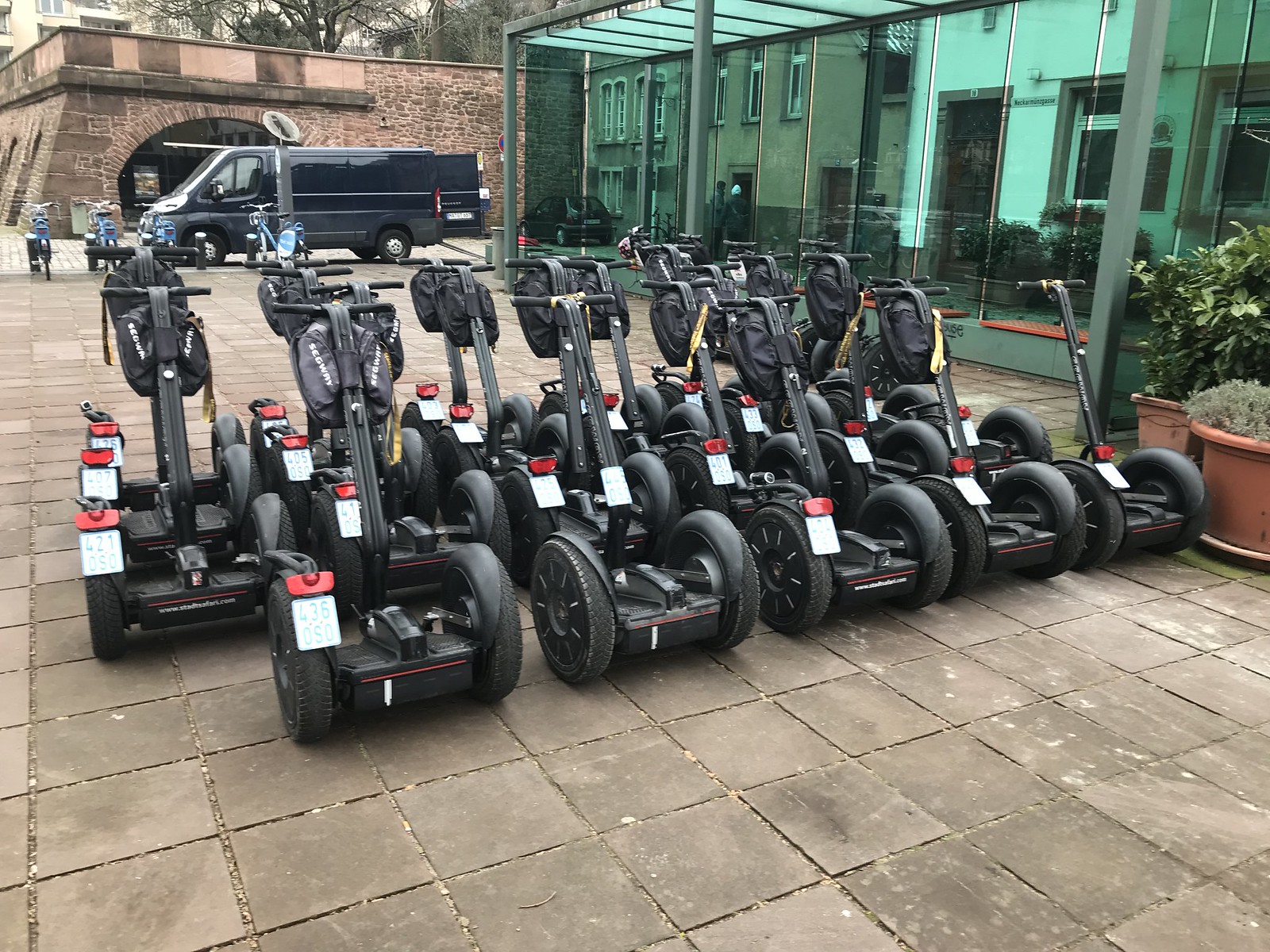The image captures a modern and minimalist one-story building with green-tinted reflective windows. Around the building, there is a covered area with a green glass awning supported by green metal pillars. On the sidewalk, which is paved with stone tiles in a grid pattern, there are three rows of motorized black scooters, likely Segways due to their design, lined up closely. Each row consists of about five scooters, mostly equipped with handlebar-mounted bags. The second scooter from the left in the front row is missing its bag. The scooters bear an indistinguishable red sticker with a white rectangle beneath it. To the right of the scooters are two large potted plants; one is square-shaped with a bushy plant featuring round leaves, and the other is cylindrical with a smaller, less detailed plant. In the background, a large dark blue truck with its back doors open is visible, facing left, accompanied by what appears to be four city bikes featuring light blue accents. Behind the truck, a brick building with an unusual shape is partially visible, and nearby, there's a reflective glass building acting almost like a mirror. Also in the distance, part of a stone building that looks like the bottom floor of a castle is visible, with a few leafless trees seen above it. The sky appears overcast, contributing to the subdued ambiance of the scene.